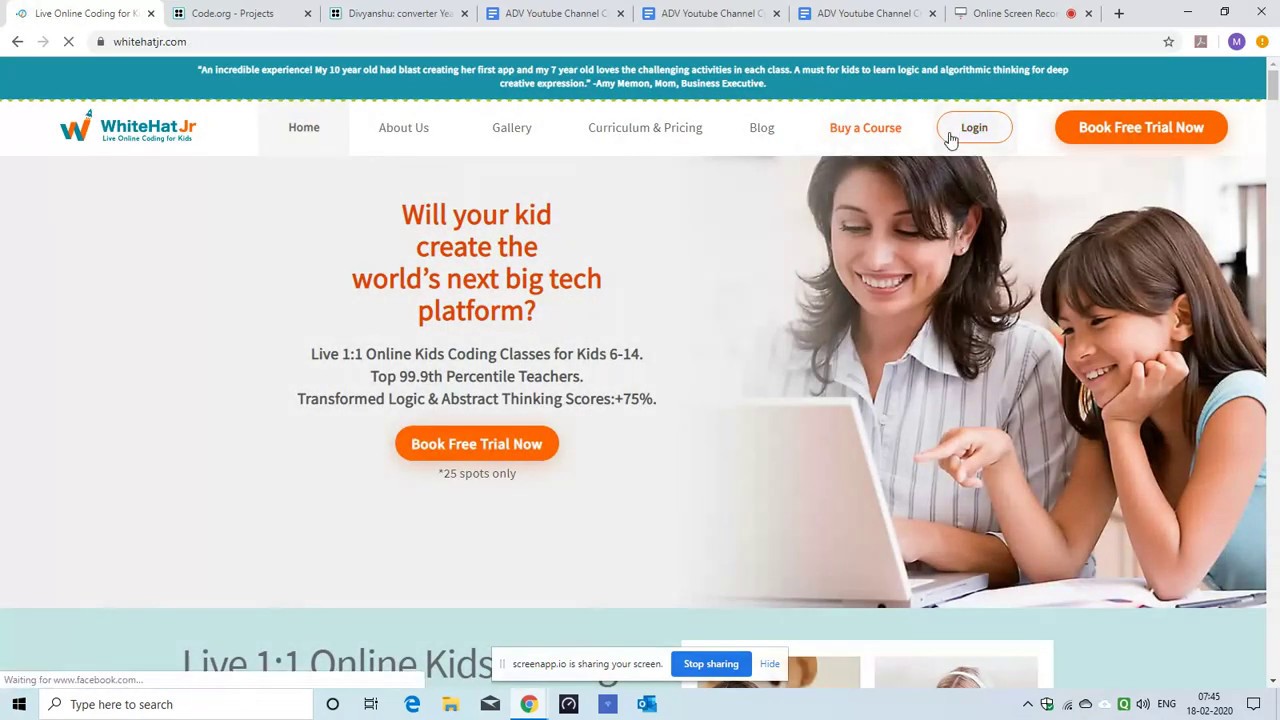An image capturing a dynamic and engaging moment in a live online kids' coding class hosted on platforms such as koe.org and the ADB YouTube channel. The scene is a snapshot of a bustling virtual learning environment filled with icons of various educational applications. A laptop screen is prominently featured with applications like Acrobat Reader and Holostar visible at the bottom. The website whitehatcher.com seems to be featured or referenced, suggesting involvement in a comprehensive coding curriculum.

In the foreground, children of ages 6 to 14 are deeply engrossed in the class, each experiencing a blend of challenge and enjoyment. One participant points excitedly at the screen, highlighting the interactive experience. The clock at the bottom left reads 45:18, indicating that the session is in full swing. The background is alive with bright orange accents, adding energy and emphasis to the educational atmosphere.

Descriptions of the curriculum reveal a focus on logic, algorithms, and creative expression through engineering and coding challenges. The image captures the essence of a transformative learning experience, where kids are encouraged to develop the skills that could drive them to create the next big tech platform. With teachers facilitating through a mix of live instruction and online resources, the image portrays a moment of innovation and discovery in the journey of young scholars.